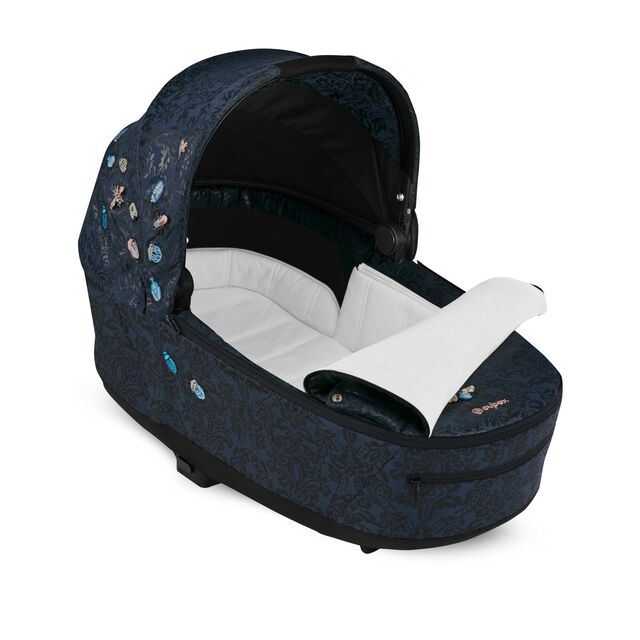The image displays a color photograph, showcasing a baby carrier designed from dark blue denim-like fabric. This portable bassinet features a cozy, white, fluffy lining inside to ensure comfort. The baby carrier is angled from the top left to the bottom right, revealing its interior. One of its notable aspects is the hood, which arches over the top left portion. The hood, lined with black felt, provides shade and protection for the baby. Along the exterior, particularly on the left side and extending to the hood, the carrier is adorned with a pattern of appliques or sewn-on decorations. Additionally, a zippered flap on the bottom right portion folds back, displaying a white underside and exposing a soft white pad with bumper rails, creating a secure and comfortable sleeping area for the baby. The photograph is set against a clean, white background, emphasizing the carrier's realistic and detailed presentation.